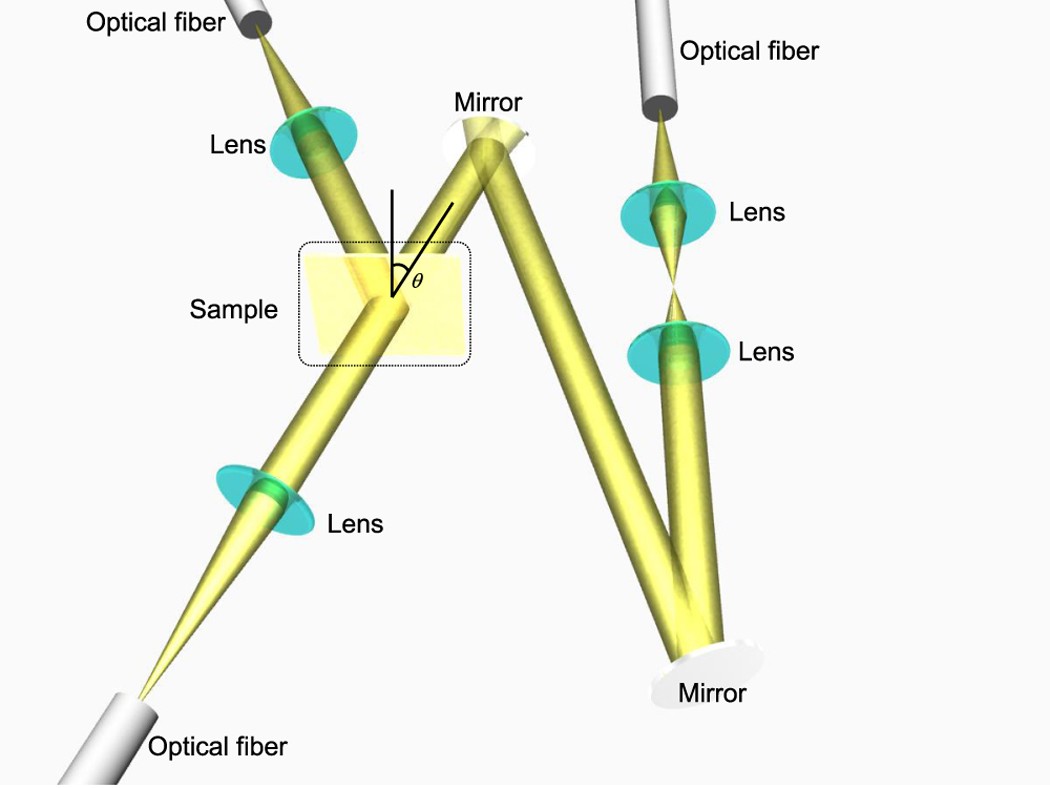In front of me is a detailed, illustrated diagram related to ophthalmology, set against a white background. The diagram prominently features multiple golden rods arranged in a W shape, intersected by a single silver rod. The labels "optical fiber" appear in the top left, bottom left, and top right corners of the image. Blue circles, labeled "lens," are positioned in three different locations along the yellow W-shaped rods, resembling contact lenses mounted on metal pipes. There are additional labels in the center, with "mirror" indicated at the convergence point of the golden rods. A small bullet box is also present, containing an upside-down "A" next to the word "sample." The color scheme includes blue, green, yellow, white, and black, suggesting the image could be AI generated or digitally drawn.